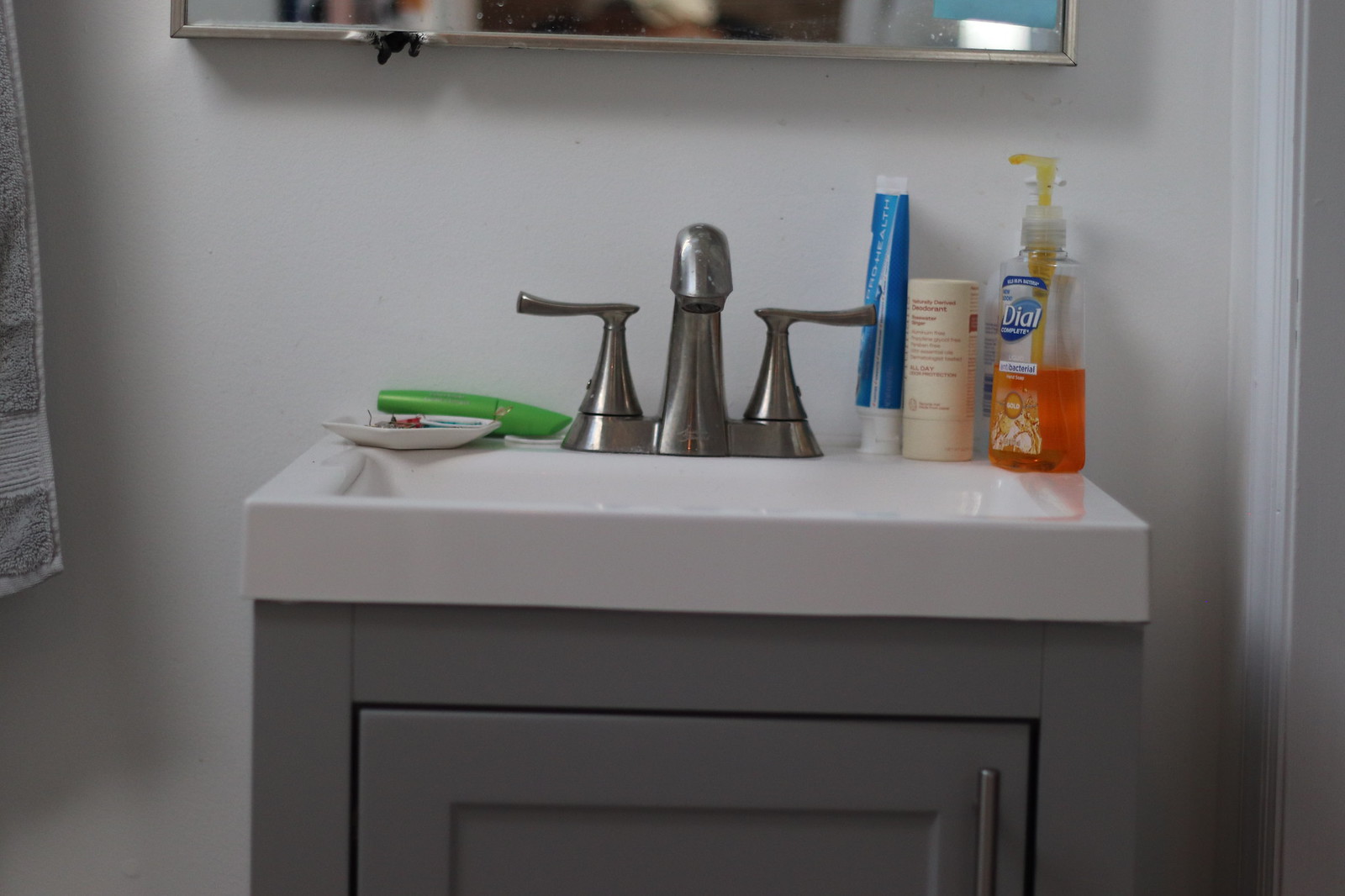The image depicts a modern, compact bathroom sink area where the sink itself is pristine white, contrasted by sleek gray cabinetry and fixtures. The chrome-colored pump faucet gleams, adding a touch of elegance to the small rectangular cabinet below. Above the sink, the bottom portion of a mirror bordered in chrome silver is visible. To the left, a towel dangles from an unseen hook, contributing to the bathroom's functionality. The walls in the background exhibit a grayish-white hue, complementing the overall color scheme. The cabinet door, designed to open to the left, features a vertical chrome bar handle on the right side. On the sink's right edge, a blue tube of toothpaste lies next to a light brown container with indistinct brown lettering. Additionally, an orange bottle of Dial hand-washing liquid with a pump dispenser is noticeable, its logo clearly displayed. To the left of the basin, a white soap dish holds a bar of soap, and a green tube rests horizontally behind it. The sink area is uncluttered and organized, showcasing a balance between modern aesthetics and practicality.